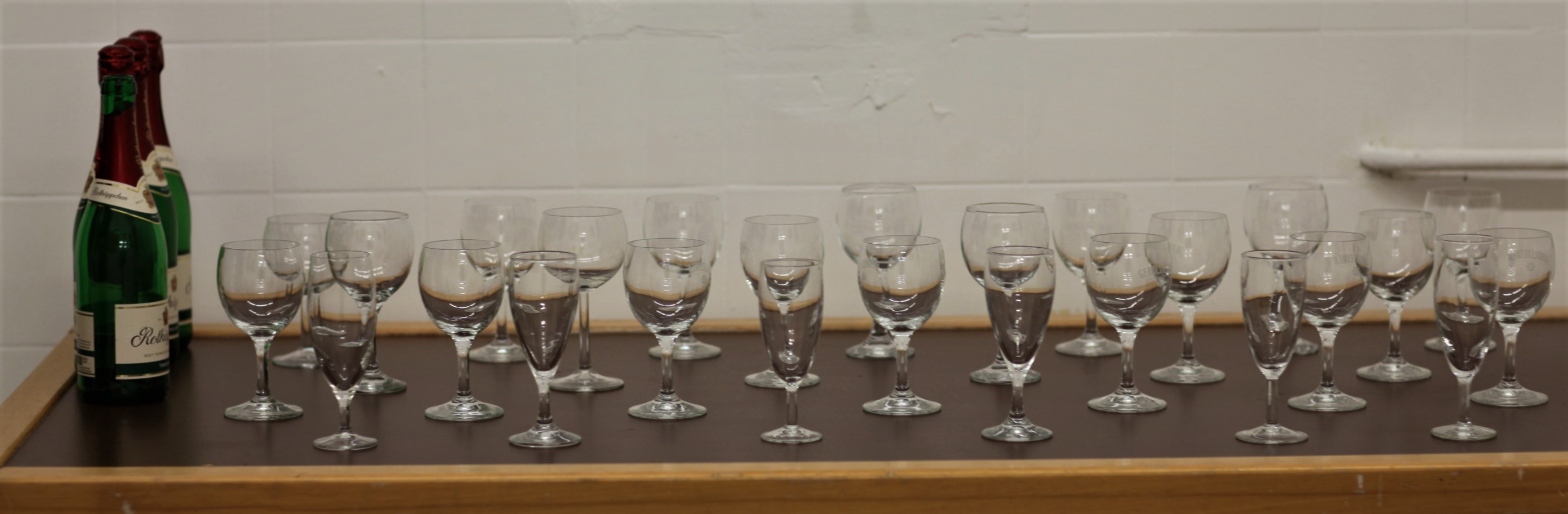In this color photograph, a dark brown table bordered with light brown edges is set against a white tiled wall. The table, possibly in a bar or similar setting, is adorned with two green champagne bottles on the left. These bottles feature red tops, white collars, and white labels with blue details. Spread across the table are approximately 25 clear glass champagne glasses, all empty. The glasses share a rounded design but vary in height, with some appearing longer in the front and shorter towards the back. Behind the glasses, a white metal rail is visible on the tiled wall. The arrangement of the glasses fills the table completely, creating an organized and symmetrical display.